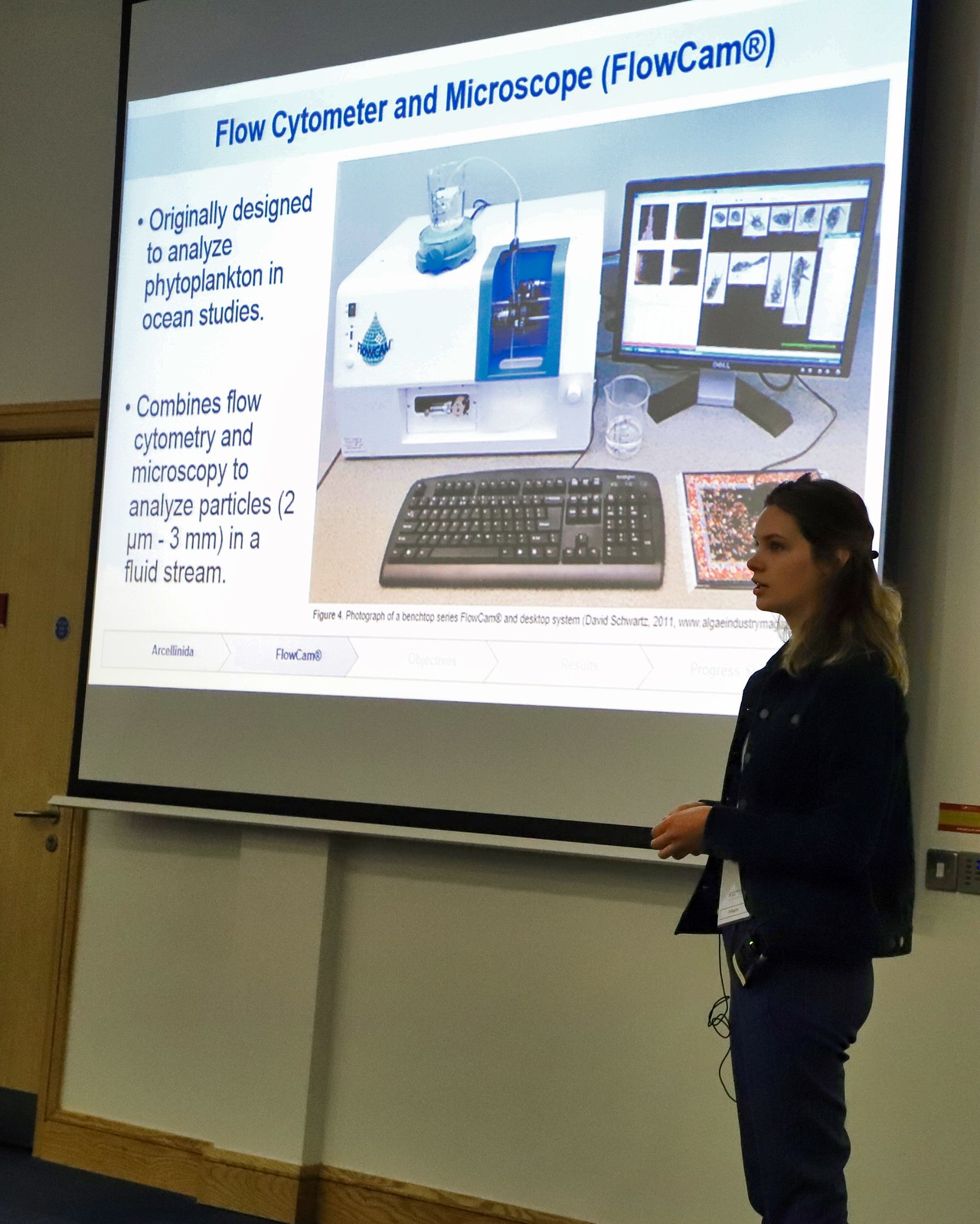The image depicts a color photograph in portrait orientation of a classroom lecture setting. At the forefront of the image, there is a woman with long dark hair pulled back, dressed in a black jacket and black pants, standing on the right side and speaking to an audience that is not visible. She is positioned next to a centrally placed projection screen. The screen displays a slide bearing the title "Flow Cytometer and Microscope" in dark blue text, with the phrase "Flow Cam®" in parentheses immediately following it. Below the title, there are two bullet points in dark blue text. The first bullet point reads, "Originally designed to analyze phytoplankton in ocean studies." The second one states, "Combines flow cytometry and microscopy to analyze particles (2mm-3mm) in a fluid stream." To the right of the text, there is a color photograph of scientific equipment, including a monitor, keyboard, and mouse, arranged in a realistic and representational photographic style. The setting and details evoke a clear and professional educational environment focused on scientific instrumentation and its applications.